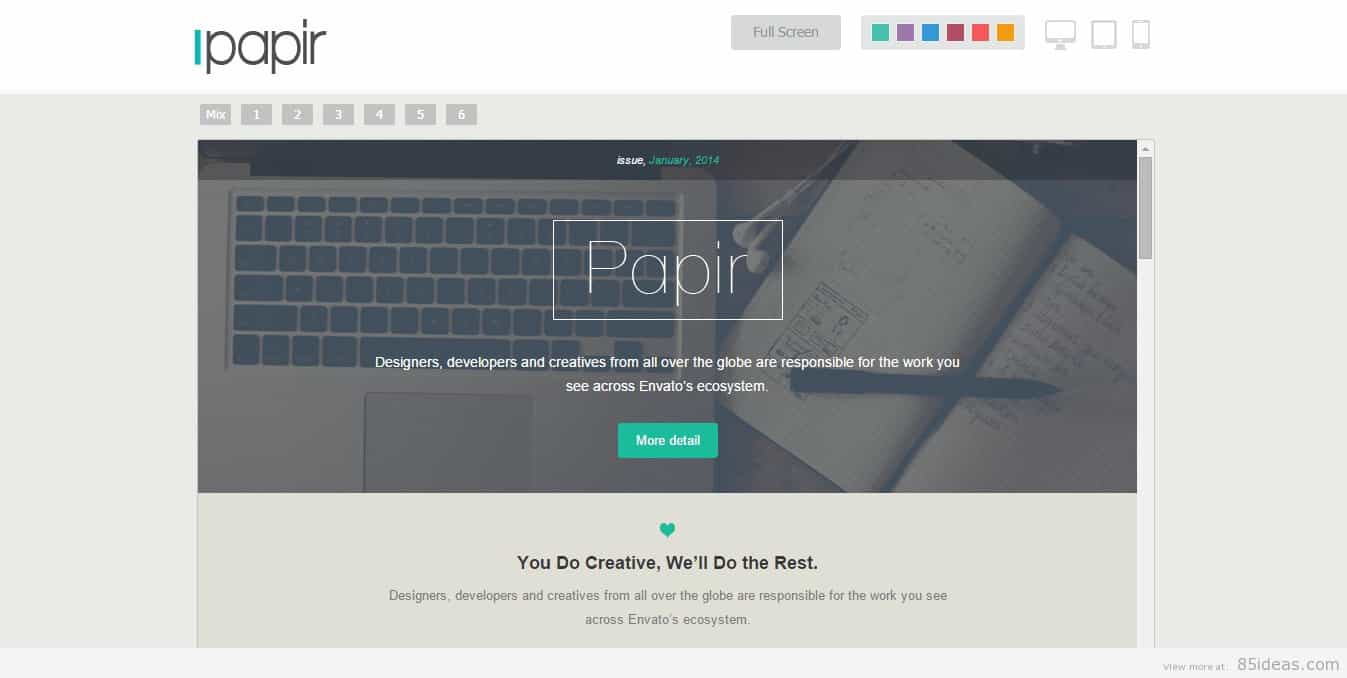This is a screenshot of what appears to be an application interface. In the upper left corner, the application name "PAPIR" is displayed in lowercase black letters, accompanied by a vertical green line immediately to the left of the first "P". The upper right corner features a gray button labeled "Full Screen" and a longer gray rectangular area filled with color squares in a sequence of green, purple, blue, red, orange, and yellow. To the far right of the color squares are gray icons representing a computer monitor, a tablet, and a cell phone.

Dominating the center of the screen is a detailed image featuring a gray computer keyboard positioned on the left side. To the right, an open notebook lies at a diagonal angle, showing pages with black handwritten text. A sleek black pen rests diagonally along the center crease of the open book. Just to the left of this pen, white text reads: "Designers, developers, and creatives from all over the globe are responsible for the work you see across Envalo's ecosystem." Directly beneath this statement is a rectangular green bar bearing the text "More Detail" in white letters. Above this bar, encased in a white-outlined box, the word "PAPIR" is capitalized.

At the very bottom of the screenshot, set against an off-white background, is a green heart icon. Below the heart, bold black text states: "You did creative, we'll do the rest." This is followed by another line of lighter black text reiterating, "Designers, developers, and creatives from all over the world are responsible for the work you see across Envalo's ecosystem."